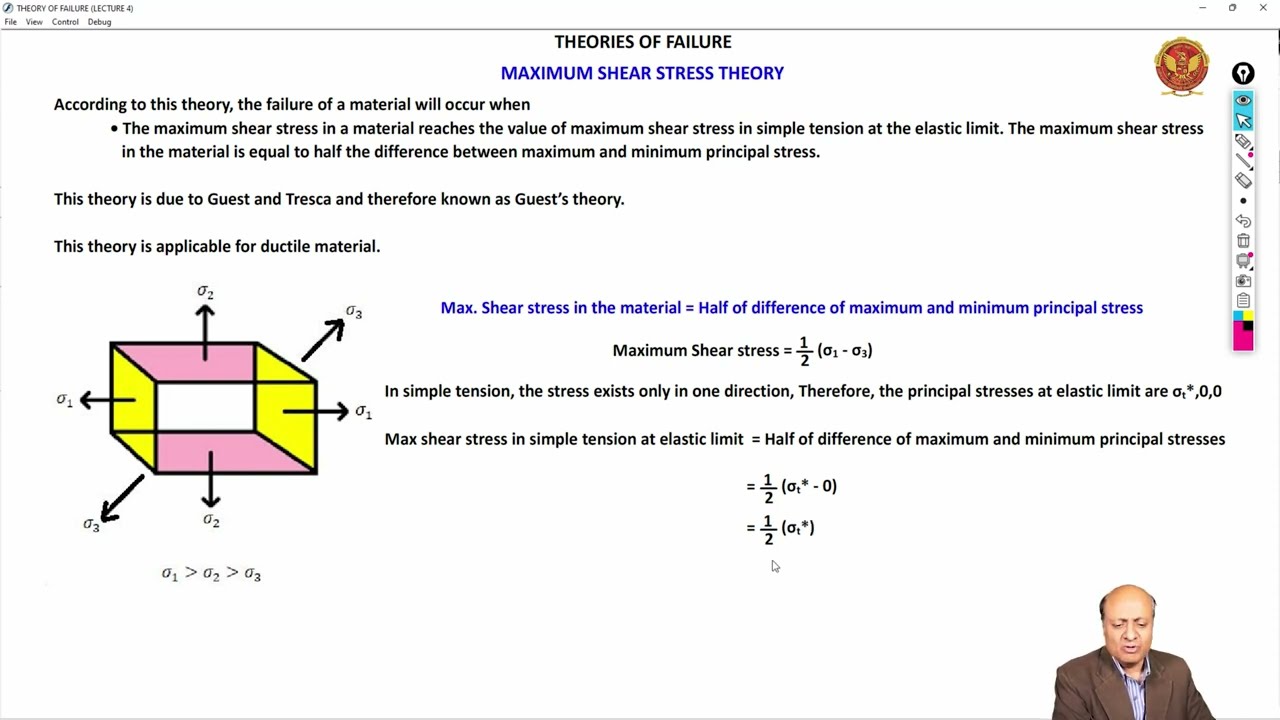The screenshot depicts an online presentation or lecture, possibly a college-level course, focused on the topic of materials engineering or theoretical mechanics. The image features an application window with a classic desktop interface, indicated by the presence of menus labeled File, View, Control, and Debug at the top-right corner.

At the top-center of the screen, in bold black text, it reads "Theories of Failure," with the subtitle "Maximum Shear Stress Theory" in blue beneath it. The central section of the screen is dominated by explanatory text detailing the Maximum Shear Stress Theory. According to this theory, failure in a material will occur when the material's maximum shear stress reaches the maximum shear stress value in simple tension at the elastic limit. This is mathematically represented by the formula where the maximum shear stress is equal to half the difference between the maximum and minimum principal stresses. The theory, known as Guest's Theory and attributed to Guest and Tresca, is particularly applicable to ductile materials. The text further elaborates on the equations and symbology used to describe these stresses.

In addition to the text, there's a detailed diagram on the left-hand side of the screen, featuring a three-dimensional cube-like prism with arrows and labels such as O1, O2, and O3, which denote principal stresses. The diagram is color-coded with a pink, yellow, and white boxed background and highlights the relationships between these stresses, showing that O1 is greater than O2, which is greater than O3.

In the lower right corner, there is an inset video of the lecturer, a balding man with light brown skin, wearing a brown suit jacket over a blue and white striped shirt. He appears to be speaking, suggesting a live streaming session, likely providing an explanation of the material on the main screen.

Overall, this detailed capture effectively conveys a complex lecture on the Maximum Shear Stress Theory, complete with supporting diagrams and real-time instruction from the presenter.